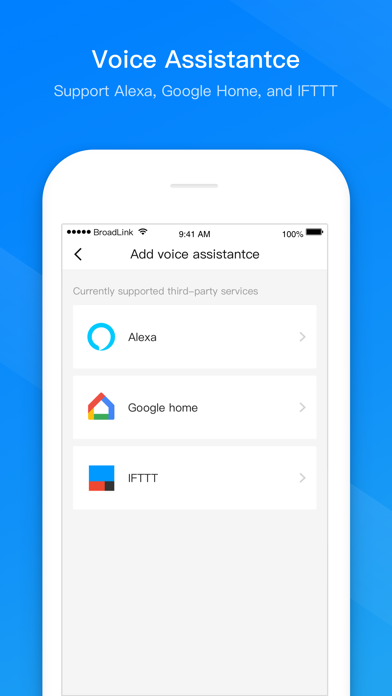The image appears to be a screenshot of an advertisement, likely positioned as a sidebar ad. It features a medium blue gradient background with a lighter blue line running horizontally through it. At the top of the ad, in white text, it advertises voice assistant support, specifying compatibility with Alexa, Google Home, and IFTTT.

Central to the image is a generic white iPhone, which could represent any iPhone model. The iPhone's screen displays a UI from Broadlink, indicating the current time as 9:41 a.m. with a full 100% battery. The screen has a simple, clean design with a white and light gray background, black text, and some medium gray text accents.

The interface shows a title bar with a back button labeled "Add Voice Assistants." Below this title, there are three distinct buttons, each with a white background, black text, and unique icons to the left. The first button features a blue background with a white speech bubble icon and the text "Alexa." The second displays a colored square, tinted with red, blue, green, and yellow, alongside the text "Google Home." The third button shows a mix of blue, orange, and black rectangles and squares with the text "IFTTT."

Overall, the advertisement aims to highlight the device's compatibility with popular voice assistant platforms.